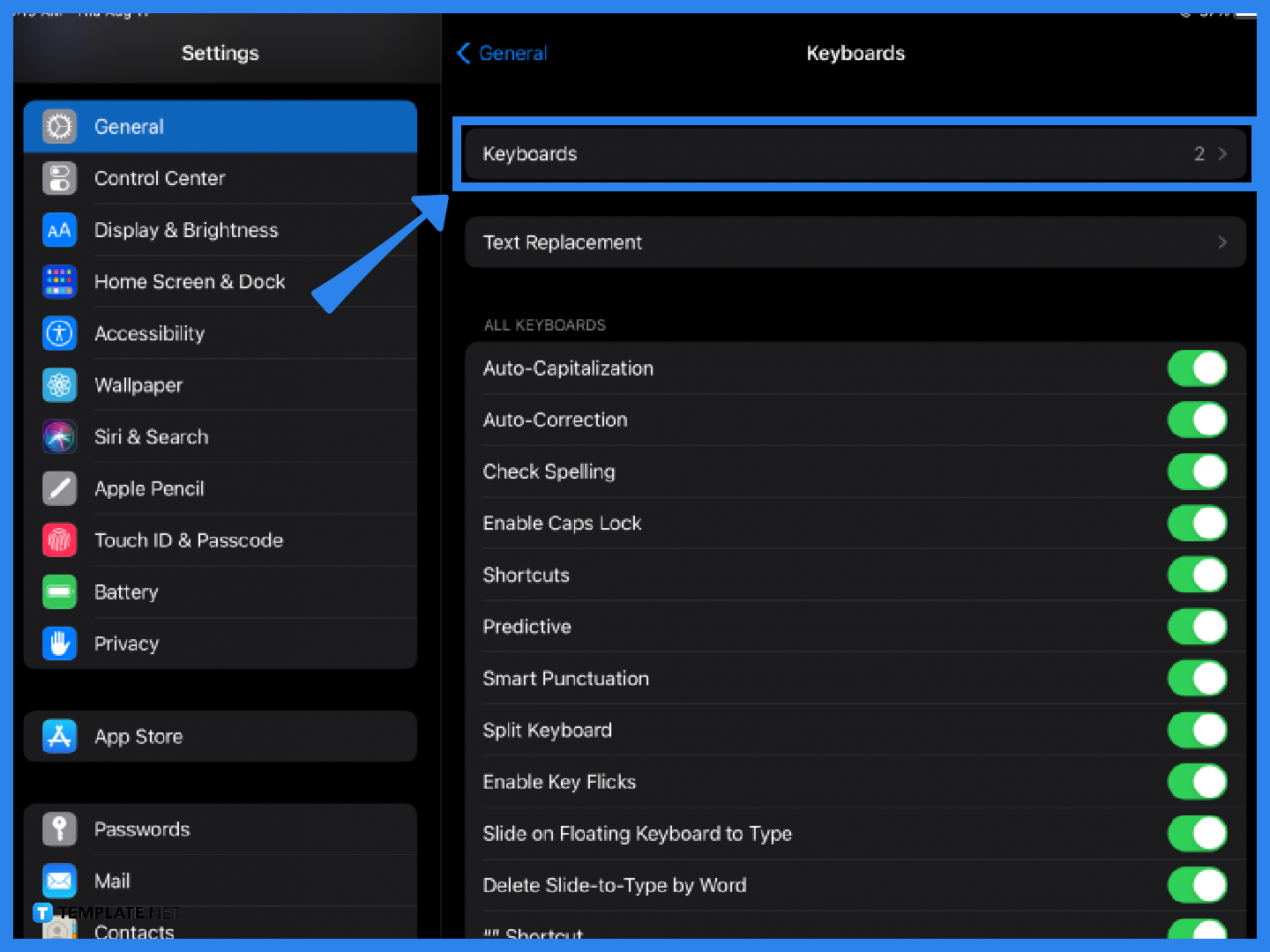This image displays a screenshot of an iPhone's "Settings" menu, specifically within the "General" section. The "General" menu option is highlighted in blue, indicating it has been selected. Within this section, there is a hand-drawn arrow pointing from the "Home Screen & Dock" tab towards the "Keyboard" tab, which has also been outlined with a blue border, directing attention to this specific area. Below "Keyboard," several sub-options are listed, including "Text Replacement." The highlighted section reveals various settings for different keyboards, each accompanied by toggle switches. The toggles are predominantly green with white switch indicators, suggesting active settings. If a switch is toggled off, it would appear grey, indicating an inactive state.